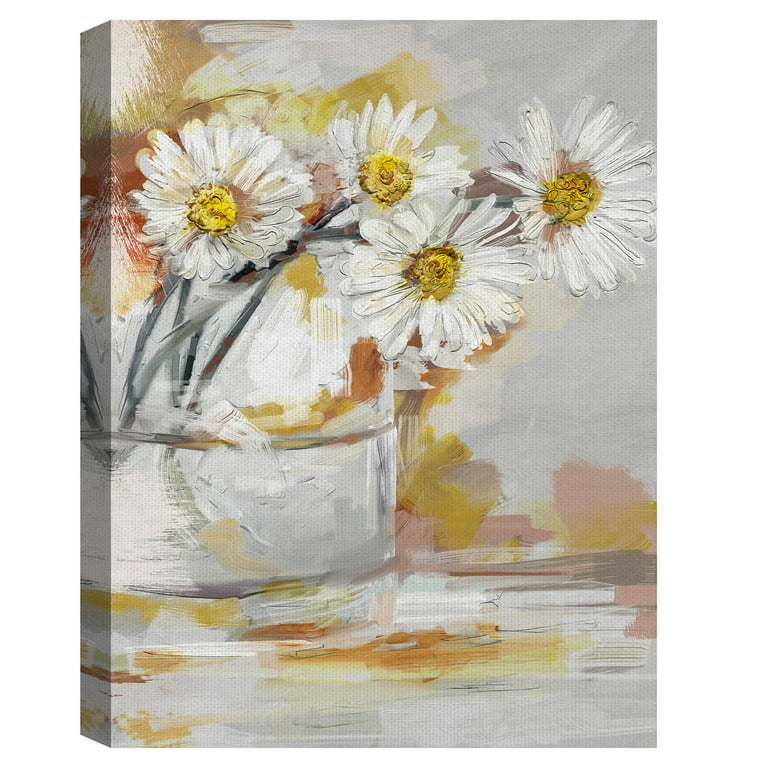This oil painting prominently features a delicate arrangement of four daisies with white petals and yellow centers, set in a translucent, see-through glass vase. The daisies' green stems gracefully extend into the vase, which is partially filled with water. The vase is short, wide, and round, resting on a textured base that combines hues of light gray, white, and hints of light pink, yellow, and orange. This same mottled and muted effect is echoed in the background, which blends gray with warm tones like gold, bronze, and rust. The entire canvas evokes a serene and soft atmosphere, with the colors smoothly transitioning and layering over each other, enhancing the ethereal presence of the daisies against the subdued backdrop.